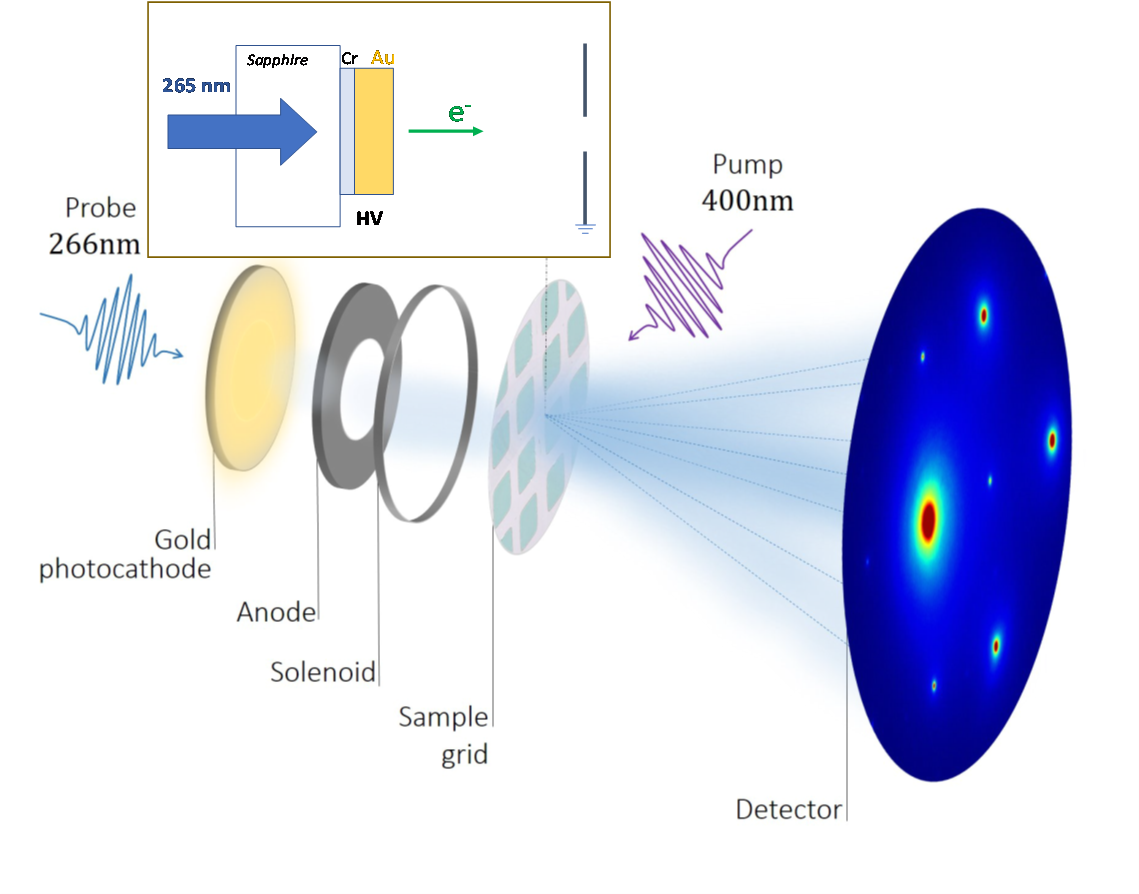The image details the functioning of advanced space telescopes and detectors, specifically akin to those on the James Webb Space Telescope. At the top, a blue arrow labeled "265 nm" points to a sapphire material, followed by a depiction of gold (AU). Below this, an intricate schematic unfolds: a blue wave indicated as "Pump 400 nm" enters the gold photocathode, a golden disc. Next, a gray donut-shaped ring, labeled "anode," surrounds the wave, followed by a thinner gray ring termed "solenoid." Adjacent to these, towards the right, is a circular sample grid represented as a silver disk with overlaying gray squares. This assembly captures waves labeled "Probe 266 nm" entering from another direction. Further right, a detector presents a blue image of outer space sprinkled with red and green areas, likely illustrating heat generٌations from stars. The visual meticulously breaks down the components and interactions within the optical and detection systems, comprising numerous disk shapes and waves, akin to what a solenoid and supporting lenses might illustrate in a detailed operational guide.